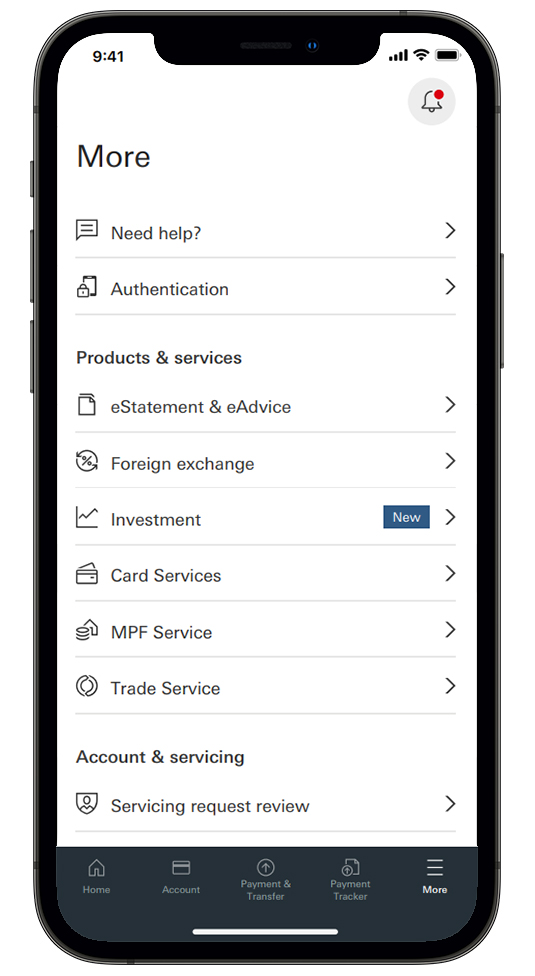The image depicts an iPhone displayed on a white background, showcasing a mobile application interface. The app screen has a dark gray menu bar at the bottom with five options arranged from left to right: Home, Account, Payment & Transfer, Payment Tracker, and More. Each option is accompanied by a corresponding icon above the label. The "More" option is highlighted in white, indicating it is currently selected, while the other options appear in light gray.

In the "More" section, the app has a predominantly white background. At the top left in black text, it says "More." Adjacent to the top right corner is a bell icon with a red notification circle. Below the title, two options are listed: "Need Help" and "Authentication," each with an arrow pointing to the right. The "Need Help" option is paired with a chat box icon, and "Authentication" is represented by a padlock and phone icon.

Further down, there is a section labeled "Products and Services," featuring several options: 
1. eStatement and eAdvice
2. Foreign Exchange
3. Investment, which has a "NEW" label in blue adjacent to it
4. Card Services
5. MPF Service
6. Trade Service

Each of these options is marked with an icon to its left – for instance, the "Investment" option is accompanied by a financial graph icon.

Continuing downward, another section titled "Account and Servicing" appears, with "Servicing Request Review" listed underneath it, complete with an appropriate icon next to it.

The meticulous detailing of icons, labels, and arrangement of menu options provides a clear and organized presentation of the iPhone app's interface.